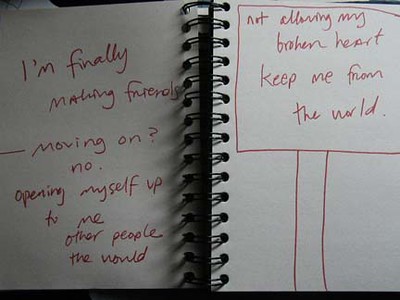The image displays an open spiral-bound notebook, held together by 15 black double rings along the spine. Both visible pages are white and unlined, with handwritten text in red ink. On the left page, the text reads: "I'm finally making friends, moving on? No, opening myself up to meet other people, the world." The right page features a reddish square with a thin vertical post beneath it, resembling a sign, containing the words: "Not allowing my broken heart to keep me from the world." All the writing is in lowercase, conveying a personal struggle and emotional journey, reflecting the intimate thoughts typically found in a journal or diary. The grammar is slightly imperfect, adding to the authenticity and rawness of the emotions expressed.